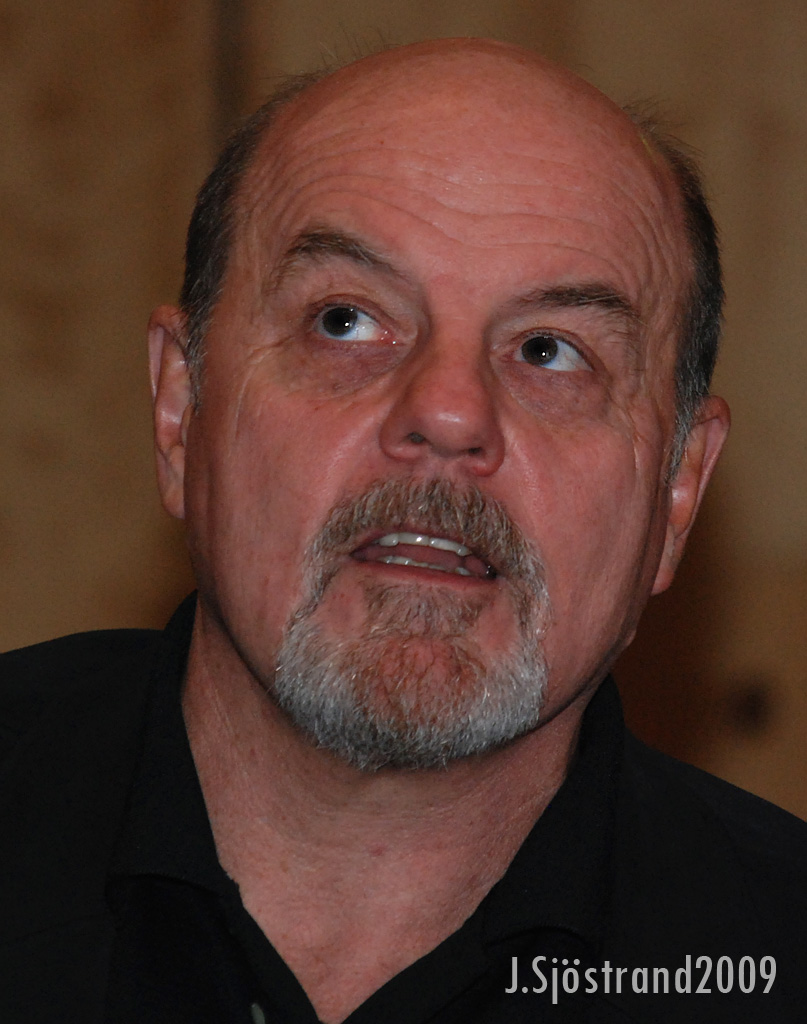The photograph is a detailed close-up of a man, visible from his upper shoulders to the top of his head. He has a receding hairline with gray hair primarily on the sides of his head. His facial hair includes a neatly trimmed gray mustache and beard, leaning towards a salt-and-pepper shade. He is dressed in a black polo shirt with the top two buttons undone. The man is looking up and to the left, suggesting a contemplative or reflective expression. His eyebrows are dark and bushy, and his eyes also appear dark. The background is out of focus and predominantly tan, providing a neutral backdrop. In the bottom right corner, the image has a watermark in white text that reads "J.S.J.O.S.T.R.A.N.D. 2009". The image style aligns with Photographic Representationalism and Realism, capturing the detailed textures and expressions of the subject.